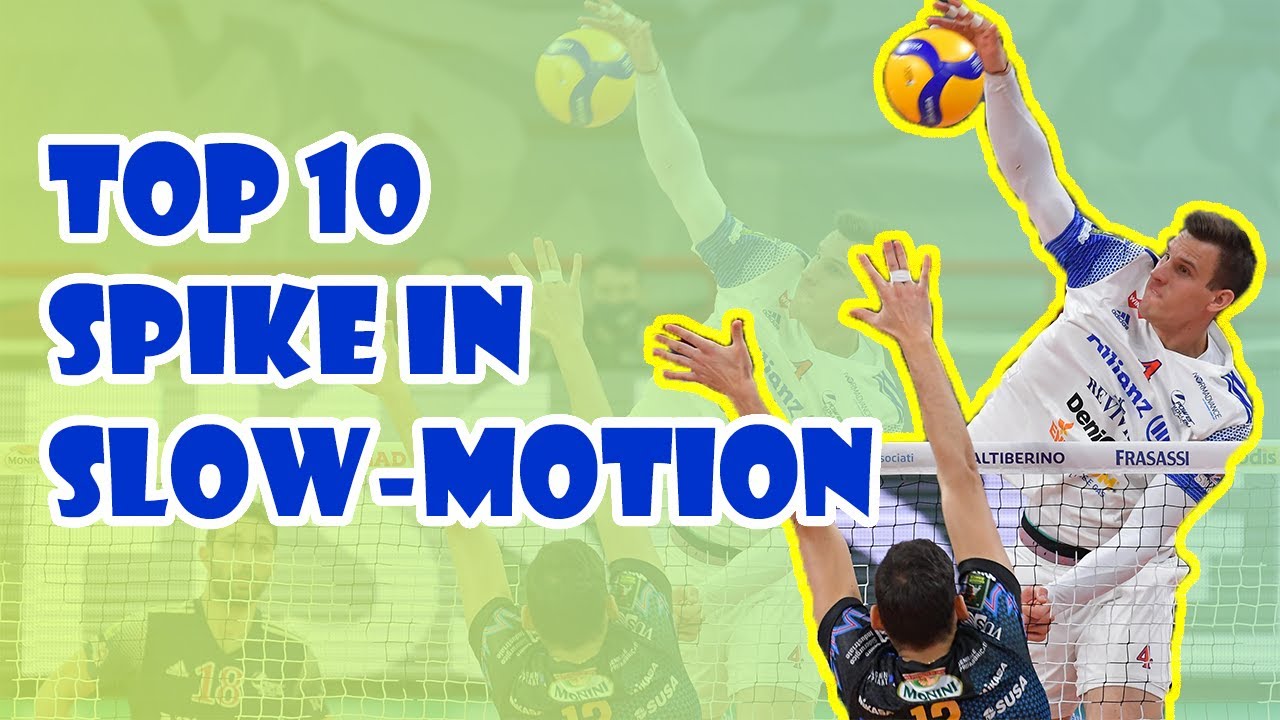The image captures an intense volleyball match in mid-action. On the right side of the frame, two players are highlighted with a yellow outline. The player in the foreground, dressed in a white uniform with blue trim, appears to be striking a yellow and blue volleyball over the net. This player is in a spiking motion, with a white net visible below him. Opposite him, another player in a darker uniform of blue and black is trying to block the spike with arms fully extended upwards. The background has a blurry greenish gradient, which also faintly mirrors the same volleyball players, adding depth to the scene. To the left of the image, in large, bold blue text with a thick white outline, the words "Top Ten Spike in Slow Motion" are prominently displayed. The text is arranged in three lines and contributes to the overall sporty layout of the graphic, suggesting that this could be a video thumbnail showcasing dramatic volleyball spikes in slow motion.